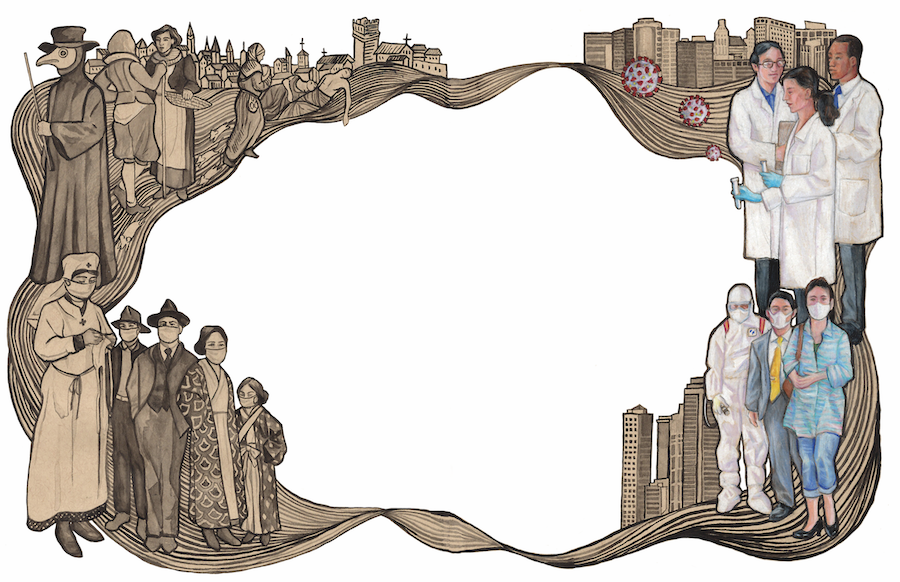The image is an animated drawing that features a border made up of various scenes related to healthcare throughout different historical periods. In the top left corner, a character dressed in a large robe, a pointy mask, and a top hat akin to a plague doctor from historical plague times is visible, representing a bygone era of medical practice. Below it, multiple individuals are depicted wearing masks and traditional outfits, possibly kimonos. The top right section shows modern healthcare workers adorned in doctor's coats, engaging with test tubes, with an abstract representation of the coronavirus floating in the air, symbolizing contemporary medical challenges. In the bottom right, three more healthcare workers in masks are portrayed with city buildings in the background, emphasizing their urban setting. The center of the image is notably blank, with all these scenes forming a cohesive border around it. The clarity of the image is high, with bright natural light enhancing the detail and vividness of each section.